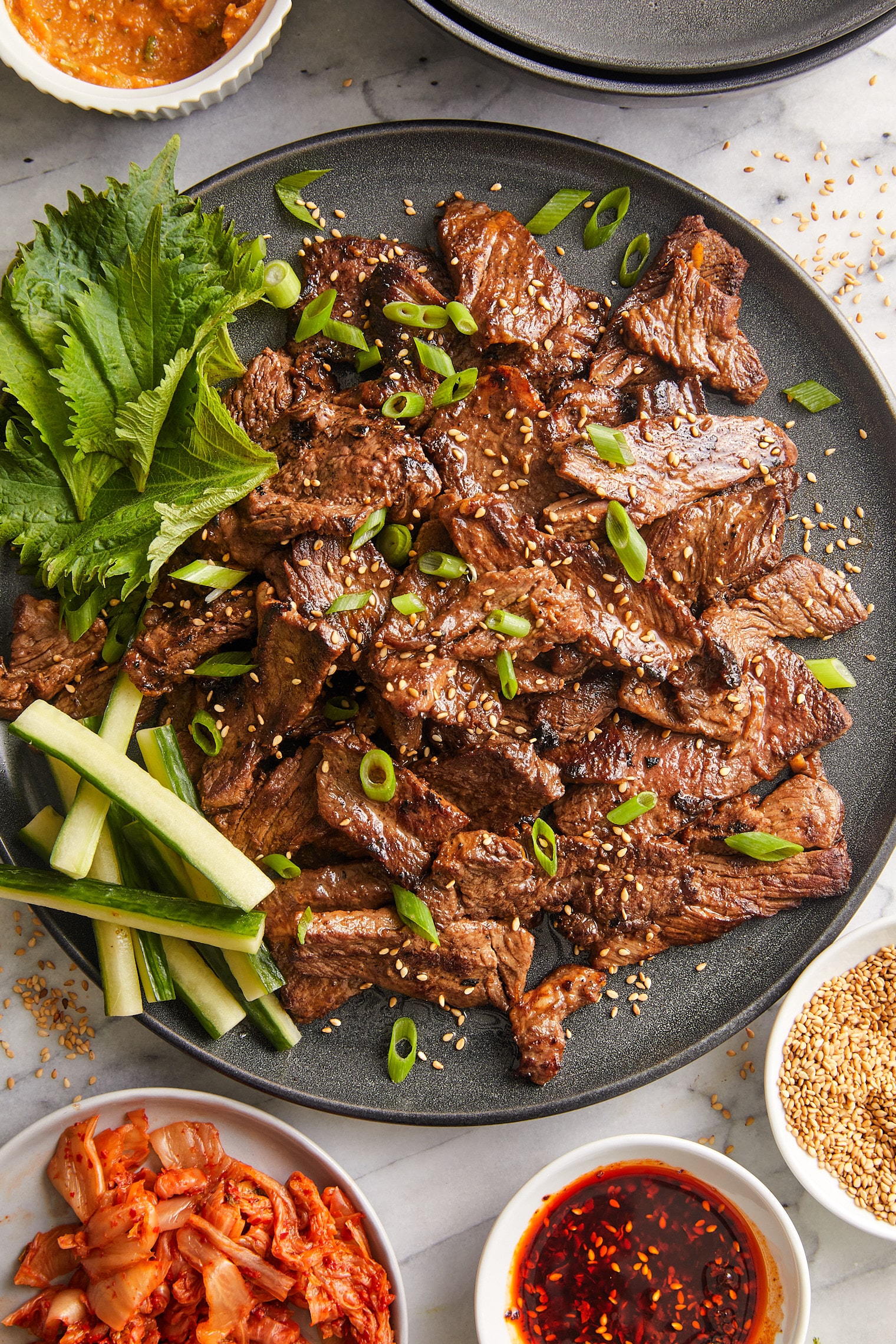The photograph appears to be a professionally styled, close-up shot of a Korean-inspired meat dish intended for a cookbook or recipe guide. The central focus is on a large, flat, gray-speckled dish laden with small, succulent chunks of beef, garnished generously with slices of green celery and green onions, along with a light sprinkle of sesame seeds. The plate also features what seems to be leafy parsley or spinach positioned just above the vegetable slices. On the left side, there is an arrangement of cucumber sticks, resembling thick-cut french fries.

Surrounding the main plate are smaller white dishes containing various sides and condiments. To the left, there's a plate of kimchi, adding a traditional fermented zest to the presentation. Adjacent to the kimchi is a white bowl with a vivid red dipping sauce, speckled with sesame seeds, suggesting a spicy or tangy flavor profile. Next to the dipping sauce is another bowl filled with what appears to be roasted sesame seeds. At the bottom of the image, there's a glimpse of a ravioli-type dish, contributing an additional layer of culinary variety. The entire setup is elegantly displayed on a pristine white marble table, exuding a modern and sophisticated aesthetic. In the very top corner, a partial view of another white bowl containing an orange dip or cooked item hints at additional tastes to explore.